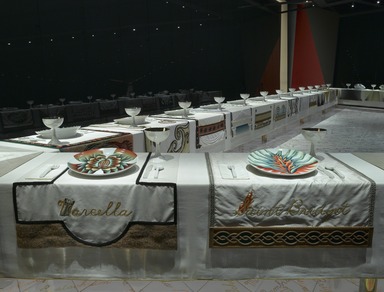The image depicts an elongated, narrow dining table draped in a white tablecloth that stretches around a corner, forming a distinctive curved setup. It evokes the arrangement you'd expect for an event, possibly a bridal party, and is devoid of any people. The foreground of the image features two ornate plates with intricate designs, one of which shows a light turquoise hue while others exhibit red, green, and blue colors suggesting floral motifs. Each place setting includes a glass and a vividly adorned plate. The tablecloth also sports gold cursive letters, but their content remains unclear due to the elaborate font. The background is dominated by a heavy, black curtain, rendering the surrounding environment indistinct and dark. A solitary white pole is visible to the right, contrasting against the otherwise dark backdrop. The floor is white, though its material is indistinguishable in the low lighting. The overall setting hints at an elaborate dinner setup, perhaps for a special occasion or a large restaurant gathering.